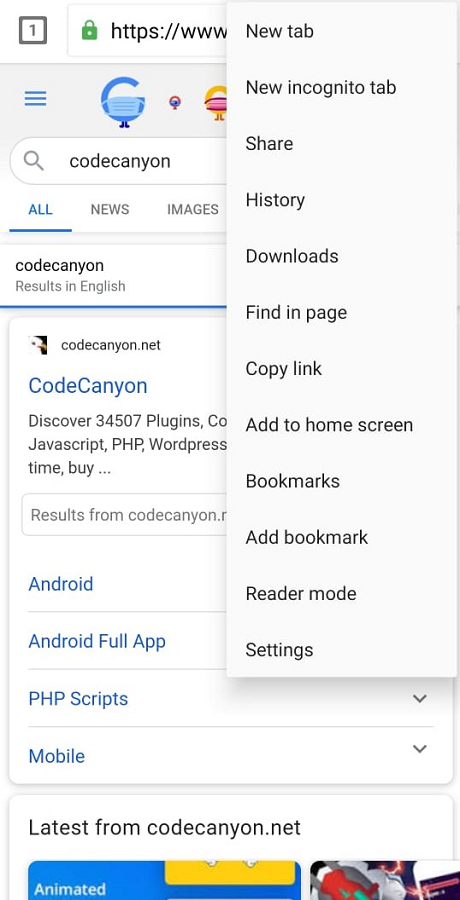This detailed descriptive caption provides a clear and precise overview of the image content:

---

The image depicts a webpage or profile page, featuring various elements and overlapping tabs. In the top-left corner, there is a square icon with the number "1" inside. Adjacent to it, partially obscured by another tab, is a search bar. The overlapping tab displays a vertical menu with several options in black text, resembling a right-click context menu in a Windows environment. The options listed are: "New tab," "New incognito tab," "Share," "History," "Downloads," "Find in page," "Copy link," "Add to home screen," "Bookmarks," "Add bookmark," "Reader mode," and "Settings."

Beneath this tab, the Google search page is visible with its recognizable layout. On the left, there are three horizontal lines (likely representing a menu). To the right, part of the Google logo is seen, but a mask covers much of it. Below the logo, the search bar contains the text "Code Canyon." The navigation options below the search bar include "All," "News," and "Images," where "All" is highlighted in blue with an underline.

Further down, search results for "Code Canyon" are displayed, starting with the text "Results in English" followed by a blue line. The top search result lists "codecanyon.net" with an accompanying icon to the left. The brief description reads: "Discover 34,507 plugins, JavaScript, PHP, WordPress," which is partially obscured by the tab mentioned earlier. Another box underneath references "Results from Code Canyon," with additional blue hyperlink options labeled "Android," "Android full app," "PHP scripts," and "Mobile." The latter two have down arrows, indicating expandable menus.

At the bottom of the image, there is a tab with the text "Latest from CodeCanyon.net" along with two images that are partially cut off.

---

This caption precisely breaks down the elements seen in the image, providing clarity on the overlapping tabs, text, and imagery.